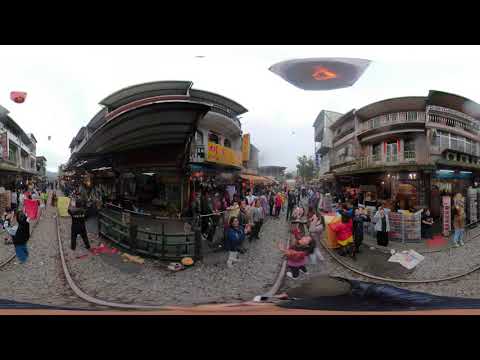The photograph captures a bustling market in a small village, possibly located in a second or third world country in Asia, suggesting an urban environment with a rustic charm. The streets, appearing rough and gravelly, are filled with a vibrant crowd, possibly between 100-200 people, engaged in various activities and possibly celebrating a festival. Colorful kites and lanterns, including pink and blue ones, float in the background against a sky dotted with three and four-story buildings that double as both storefronts and dwellings. The market streets, devoid of cars, are lined with closely packed buildings adorned with advertisements. The scene is slightly marred by visual artifacts and a gray glob with a red center, hinting at the panoramic shot's blurriness. Overall, the lively atmosphere is accentuated by people dancing, running around, and mingling in this festive, communal setting.